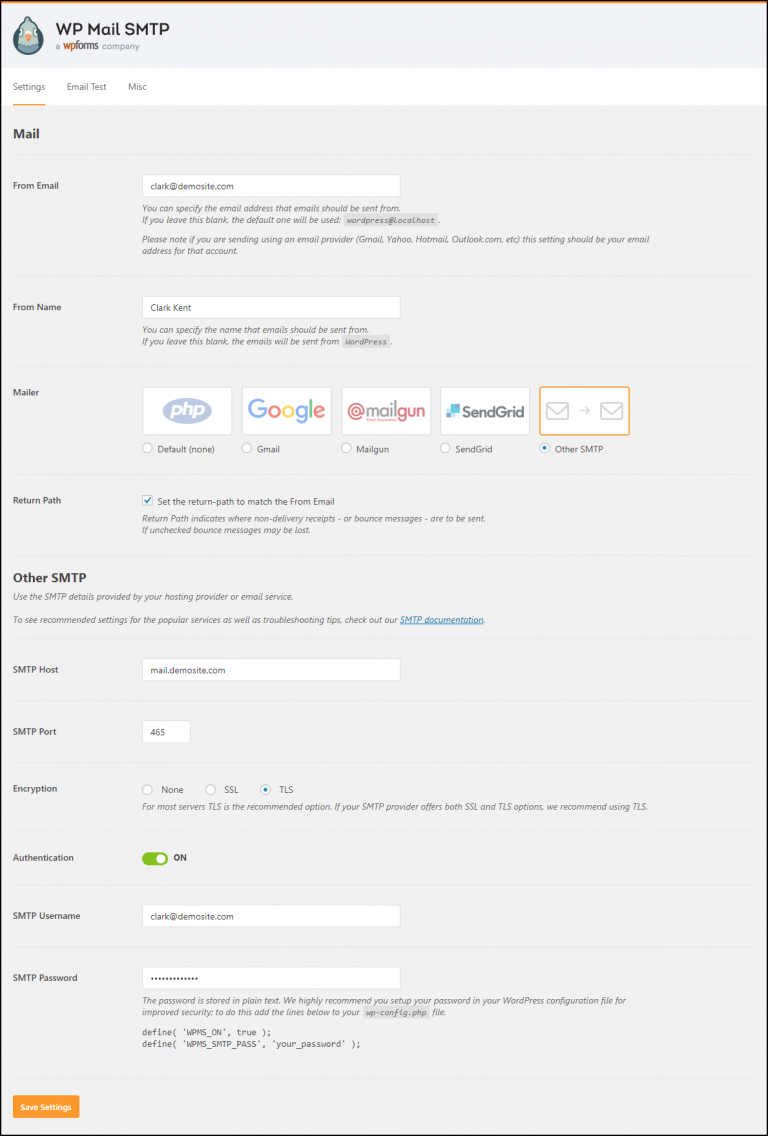The image depicts a vertically oriented screenshot resembling a tablet interface, featuring a distinct layout. The outer border is black, enclosing a light gray interior. At the very top, there's a blue-tinted bar containing a logo or icon, with colors predominantly featuring shades of teal and orange. Adjacent to the logo is the title of the site accompanied by a subtitle or description.

Beneath the top bar, a white navigation bar hosts three tabs, though the text on them is indistinct due to the sizing. The leftmost tab is highlighted with an orange underline, indicating it is the current selection. Below this navigation bar, the word "Mail" is visible, followed by smaller, illegible text.

The main content area includes a prominent white input box designated for typing, followed by a paragraph of information, and another box featuring additional information. On the left side, there is more text, which leads into a horizontal row of five emblems. The first emblem appears to represent PHP with a blue circular logo, followed by logos for Google and Magellan. The details of the remaining two emblems are unclear, though the rightmost one is outlined in orange, indicating its selection.

Continuing down the screenshot, the layout remains consistent, presenting more input boxes for typing. A notable component is a green-colored toggle switch set to the 'on' position.